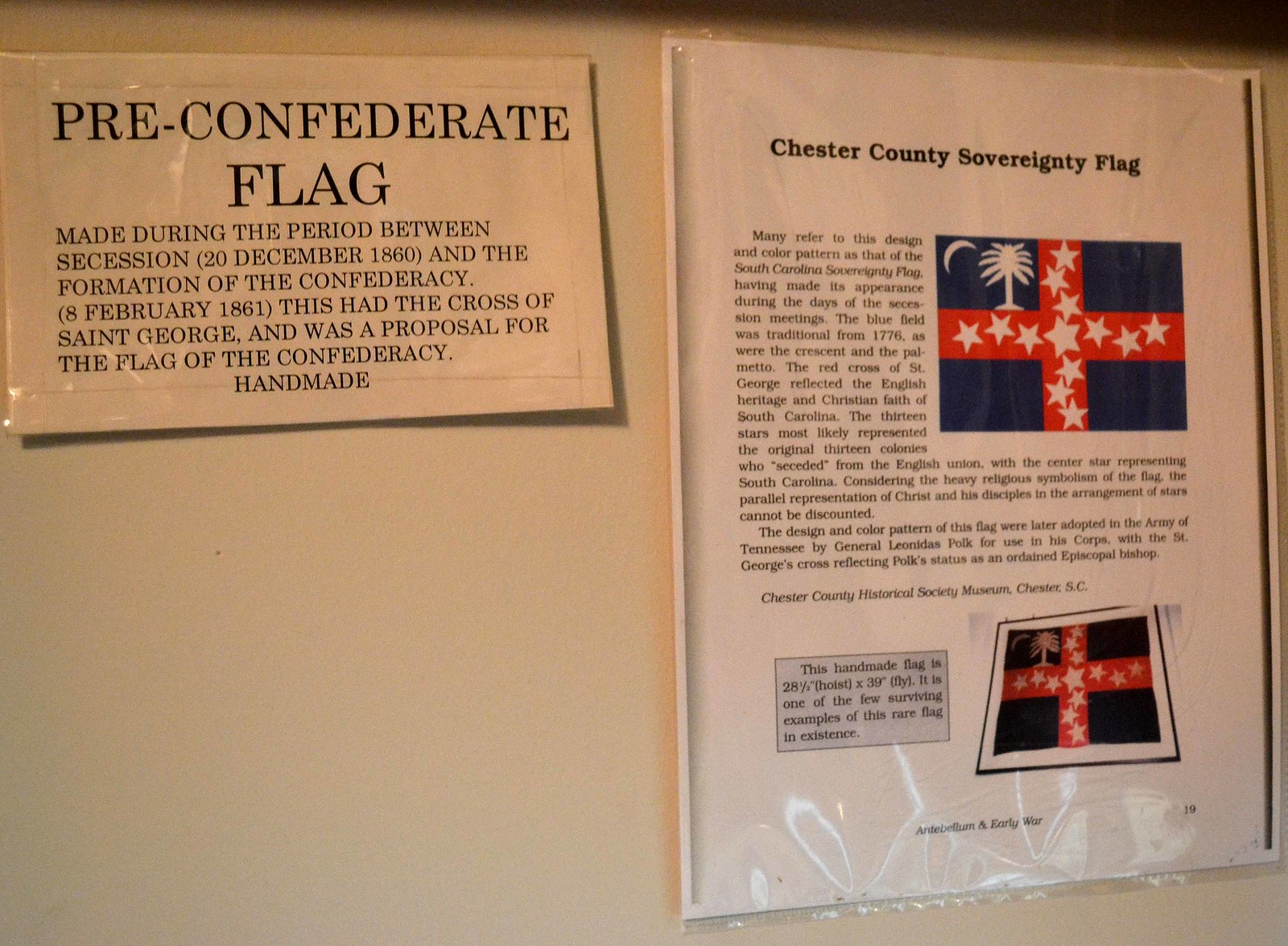The image features two pieces of laminated paper mounted on a solid white painted wall. On the left side, there is a small rectangular laminated paper containing black text. This text details the "Pre-Confederate Flag," noting that it was created during the period between South Carolina's secession on 20 December 1860 and the formation of the Confederacy on 8 February 1861. The flag included the cross of St. George and was a handmade proposal for the Confederate flag. 

To the right, a larger 8 by 11 rectangular laminated sheet has multiple lines of black text accompanied by pictures of flags. This text describes the "Chester County Sovereignty Flag." It elaborates that many refer to this design and color pattern as the South Carolina Sovereignty Flag, which appeared during the secession meetings. It mentions that the blue field was a traditional choice dating back to 1776. The sheet includes detailed explanations and images of the flags, with one image featuring a red cross horizontally set against a blue background with a palm tree in the upper left quadrant.

The overall presentation resembles an official plaque, emphasizing the historical context and visual details of these significant flags.